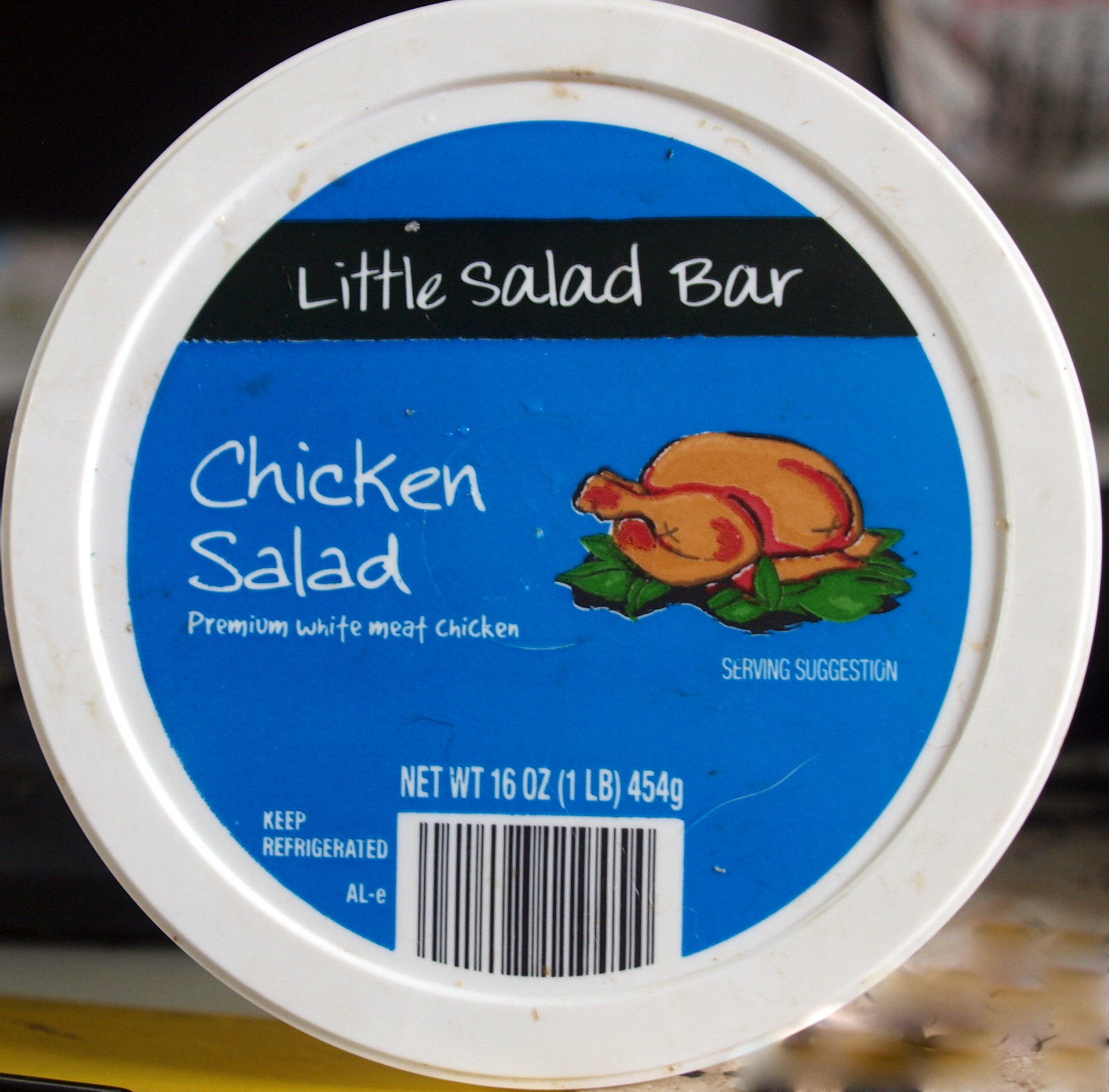This is a detailed close-up photo of a pre-made chicken salad container from the Little Salad Bar brand. The container, lying on its side on a wooden table, prominently displays its lid. The lid features a white plastic design with a central bright blue circle, which easily captures attention. At the top of the circle, a black strip bears the brand name "Little Salad Bar." Below this, in white script, it reads "Chicken Salad, Premium White Meat Chicken." An artistic rendering of a roast chicken or turkey, plated on a bed of leaves, is depicted as a serving suggestion, although it's more illustrative than practical. The lid also includes important product information such as a large barcode at the bottom, "Keep Refrigerated" to the left of the barcode, and the weight, which is specified as 16 ounces or 454 grams, running along the top of the barcode. The image is slightly blurry on the right side and the background, providing a clear focus on the product itself.